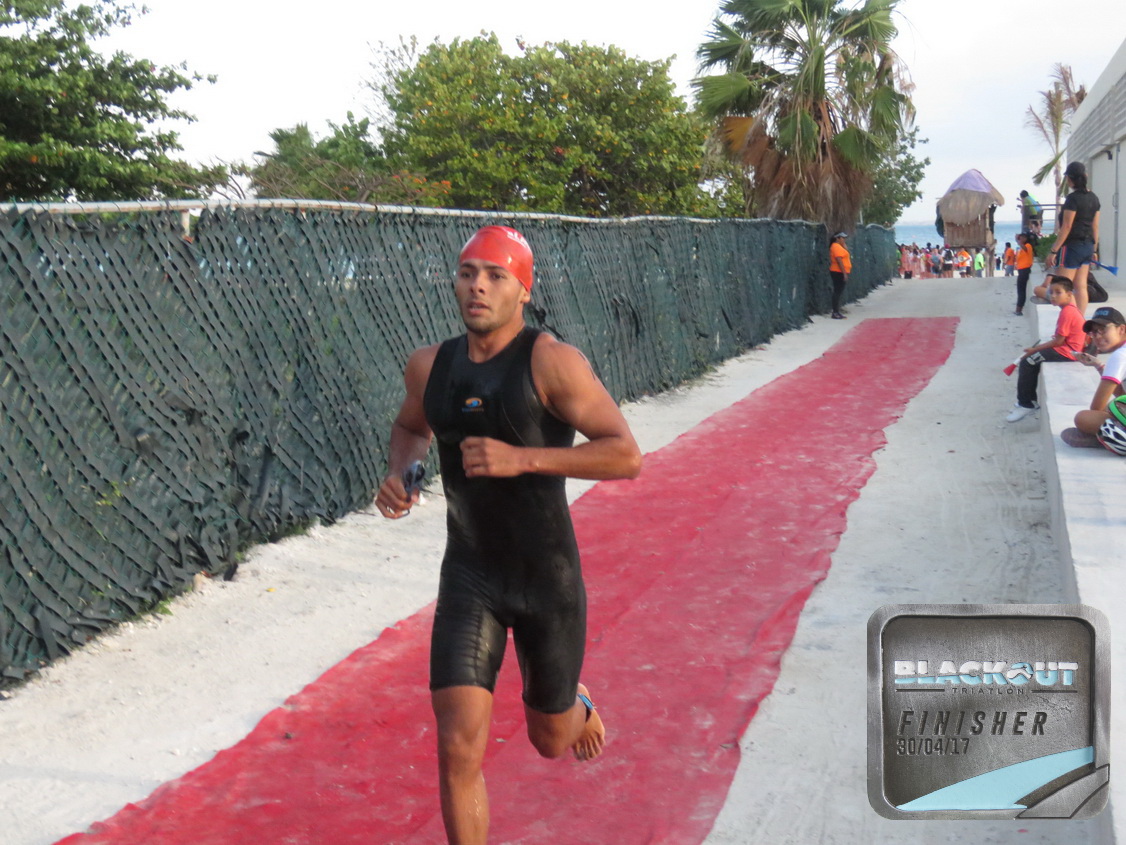This outdoor photograph captures a striking scene of a barefoot, dark-skinned man running towards the camera along a red carpeted path, possibly marking a finish line, which extends through a sandy area. The man is wearing a red do-rag, a black wetsuit, and sandals. The path is bordered on the left by a green mesh fence, behind which lush trees, including a distinctive palm tree, are visible. On the right side, a stone curb hosts onlookers, both children and adults, some seated and standing. Further in the background, a thatched-roof pavilion on stilts is encircled by people, adding to the tropical ambiance. Officials in orange shirts and casual observers populate the scene. The sky above is overcast, casting a soft, diffused light across the vibrant, modern setting. A small detail, "blackout finisher 30," is noted on the bottom right, along with the date 4-30-17, hinting at a recent event.